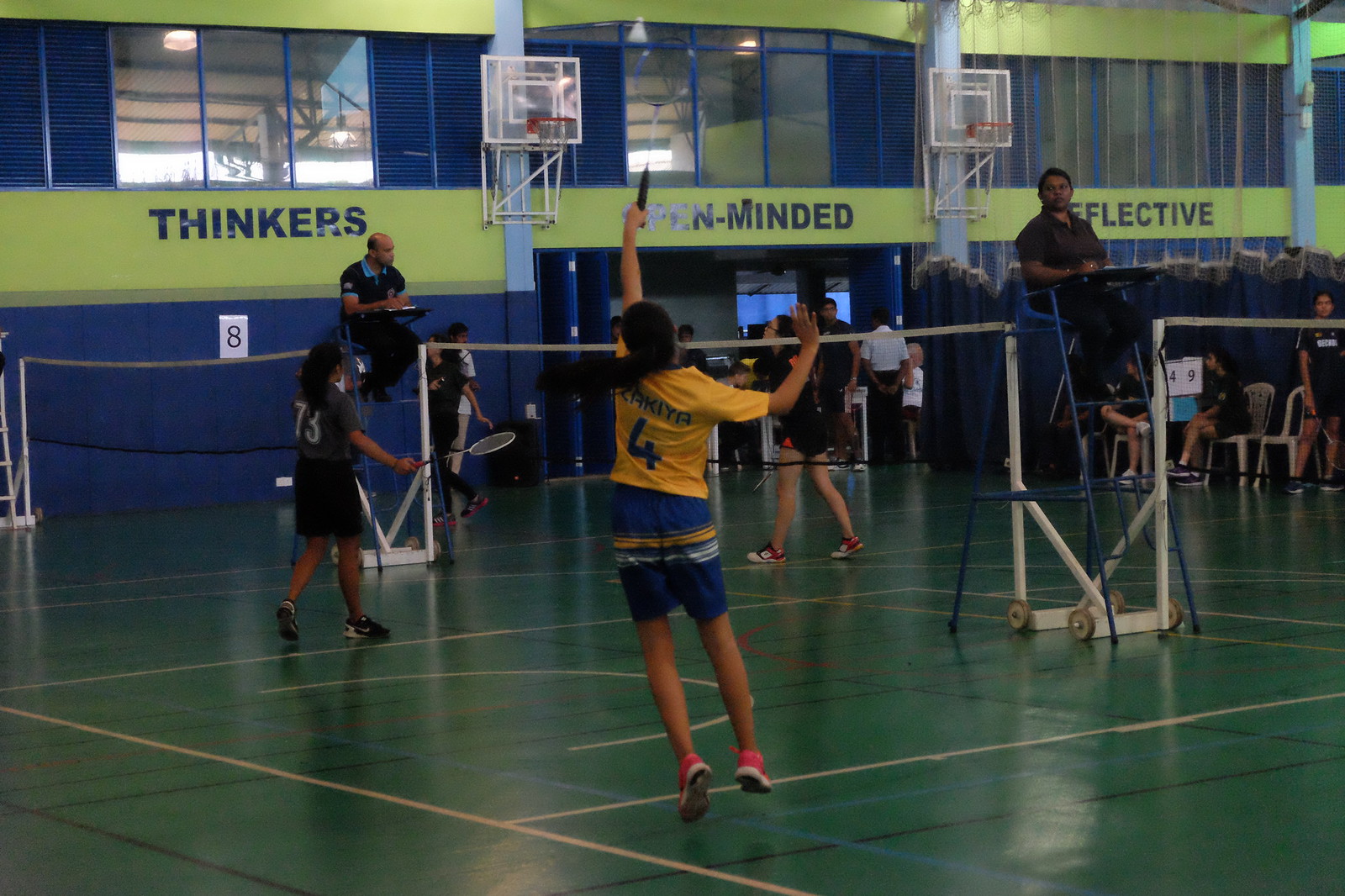In this detailed photograph of an indoor badminton court, the vibrant scene is set against a backdrop composed of green and blue walls adorned with inspirational words: "Thinkers," "Open-Minded," and "Reflective." The girl at the center of attention, clad in a yellow jersey with a blue number four and blue shorts featuring yellow and white accents, is poised to smash the shuttlecock with her racket raised high above her head. She leaps into the air, her orange sneakers visible against the dark green floor marked with various sports lines. Across the net, players in gray jerseys with white numbers prepare to respond. Above them, basketball hoops are tucked away, while two referees observe from high blue chairs. The gym is bathed in natural light from the upper-level windows, contributing to the dynamic and energetic atmosphere of multiple simultaneous matches, as wheels and onlookers frame the scene on all sides.